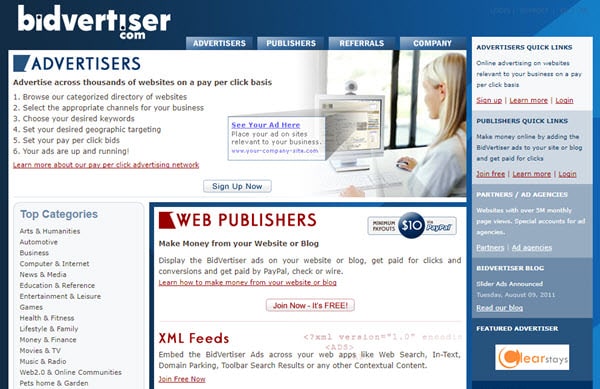The top left section displays various key terms related to online advertising, including "bid," "advertiser," "advertisers," "publishers," "referrals," and "company." A prominent white square contains the text "Advertise," along with quick links for "Online advertising," explaining the concept of advertising on websites related to your business on a pay-per-click basis. 

Highlighted in red are calls to action such as "Sign up," "Learn more," and "Login" for advertisers and publishers. For publishers, quick links include instructions on earning money online by adding the bid advertiser ads to their sites or blogs, with opportunities to join for free, learn more about the program, and login.

The section dedicated to partners emphasizes partnerships with websites that generate over 3.5 million monthly page views and details special accounts for agencies. Headings allow users to choose roles like advertiser or blog publisher, with options to utilize slider ads or announce promotions.

Detailed advertiser instructions include displaying ads across thousands of websites on a pay-per-click basis. Users can select their business category, desired keywords, and geographic targeting, and then set their pay-per-click rate to start earning money.

A segment illustrates the benefits of participating in the pay-per-click advertising network, describing how users can see their ads appear and place ads on related business sites. 

Listing top advertising categories such as "Automotive," "Business," "Computers," and many more, the section engages a wide range of industries, providing diverse ad opportunities. 

Red text highlights for web publishers include ways to make money from websites or blogs by displaying bid advertiser content, encouraging conversion to pay-per-click, and offering detailed project or wire instructions. 

Finally, users are guided on how to react, sell, feed, submit, live advertise, and ask questions, particularly for websites involving web searching, text domain parking, and contextual content.